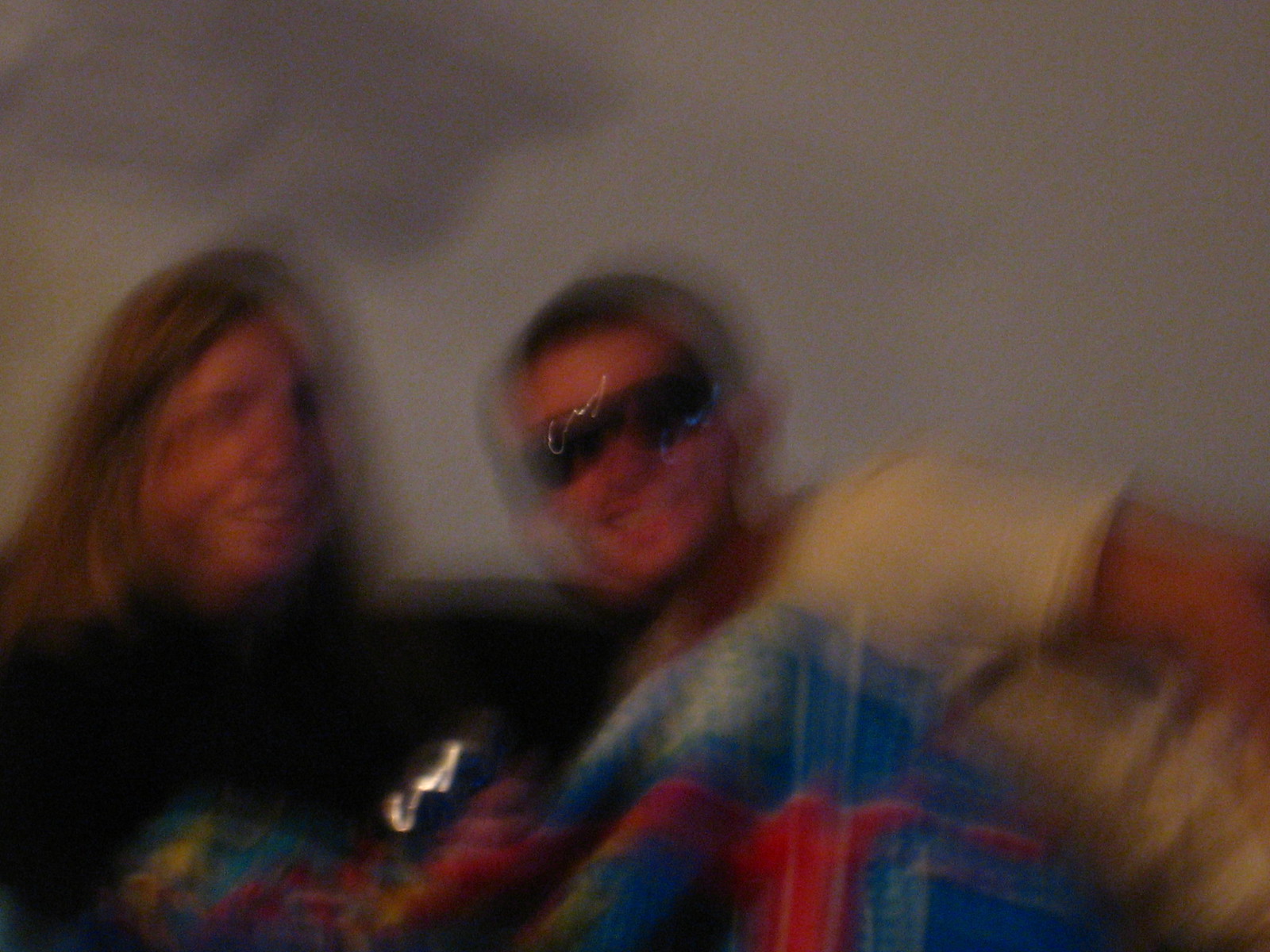In this very blurry, slanted selfie, two light-skinned individuals are posing against a white wall. The male, with short cropped dark hair and wearing sunglasses, is dressed in a yellow short-sleeved shirt. He’s leaning forward, smiling broadly with his teeth visible. The female, with shoulder-length blonde hair, is dressed in a darker high-necked shirt and has her mouth slightly open in a smile, her teeth showing. She appears to be holding a chocolate bar and is partially covered by a plaid blanket in shades of blue, red, white, and yellow, which is draped over her legs. They’re both sitting close together, with the male leaning over the female, and are bathed in shadows cast by their heads and shoulders. Despite the image's heavy blurring and shakiness, their direct gaze into the camera and clear smiles convey a moment of shared joy.